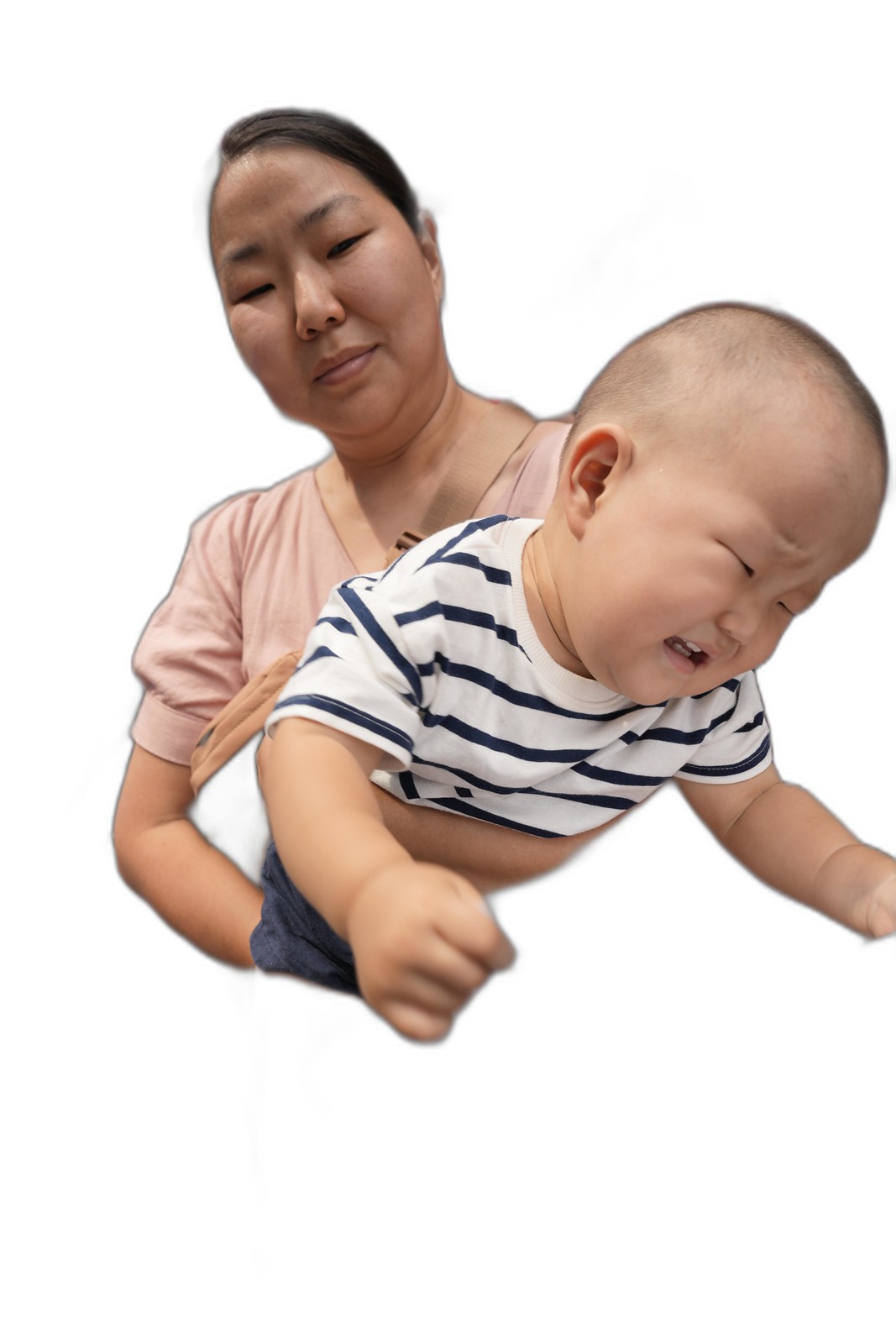In the image, a woman who appears to be Asian and around 30 years old is holding an Asian baby, possibly under a year old. The woman, dressed in a beige-pinkish blouse with a purse strap over her shoulder, is holding the baby awkwardly, with her arm wrapped around his stomach. The baby, who has a shaved head and is dressed in a navy blue and white striped shirt along with what looks like jean shorts, is crying with his eyes closed, forehead furrowed, and arms outstretched. The woman looks calmly and somewhat indifferently at the baby. The scene has a plain white background, possibly edited to remove any objects, giving the image a slightly blurred edge and an odd, almost AI-generated quality.